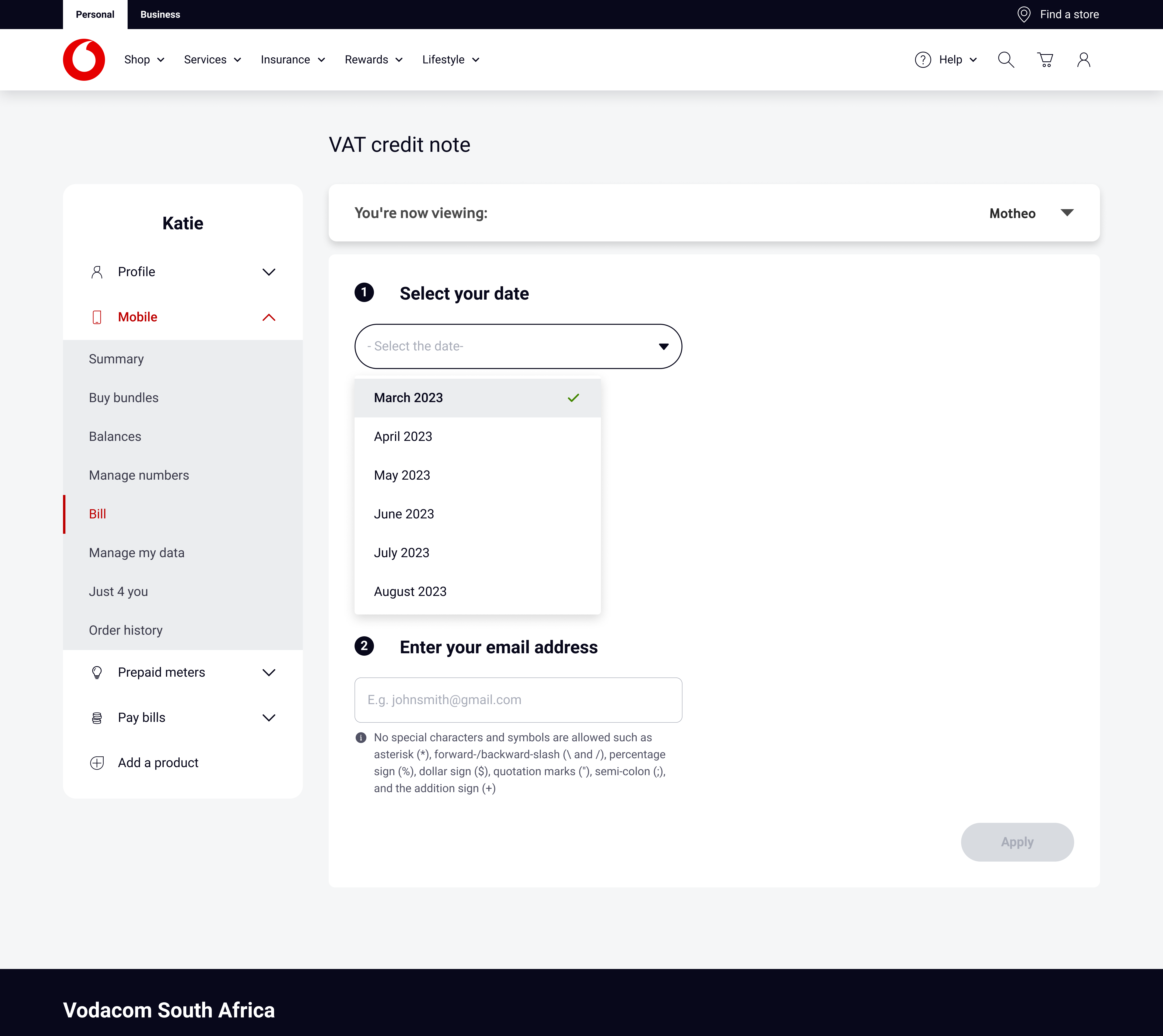This is a detailed screenshot of a web page featuring a structured layout with a prominent navigation bar at the top. The topmost section is a long, black bar with white text. On the left side, "Personal" is highlighted, indicating it is selected. To its right, additional options are "Business" and "Find a Store," both in white lettering. Directly beneath this is another bar, white in color, with a red circle containing a white comma at the far left. This bar includes drop-down menus for "Shop," "Services," "Insurance," "Rewards," and "Lifestyle." On the far right of this bar are icons for "Help" (with a question mark inside a circle), a magnifying glass (search icon), a shopping bag, and a user profile symbol.

Further down the page, centered text reads "VAT Score, V-A-T, Credit Note." On the left side, a section labeled "Katie" includes multiple drop-down options such as "Profile," "Mobile," "Summary," "Buy Bundles," "Balances," "Manage Numbers," "Bill," "Manage My Data," "Just For You," "Order History," "Prepaid Meters," "Pay Bills," and "Add a Product."

To the right of the VAT Credit Note, the text reads "You're Now Viewing," followed by "Select Your Date" and a drop-down menu offering monthly options from March 2023 through August 2023. Beneath this is a prompt to "Enter Your Email Address" with an open box for the email input.